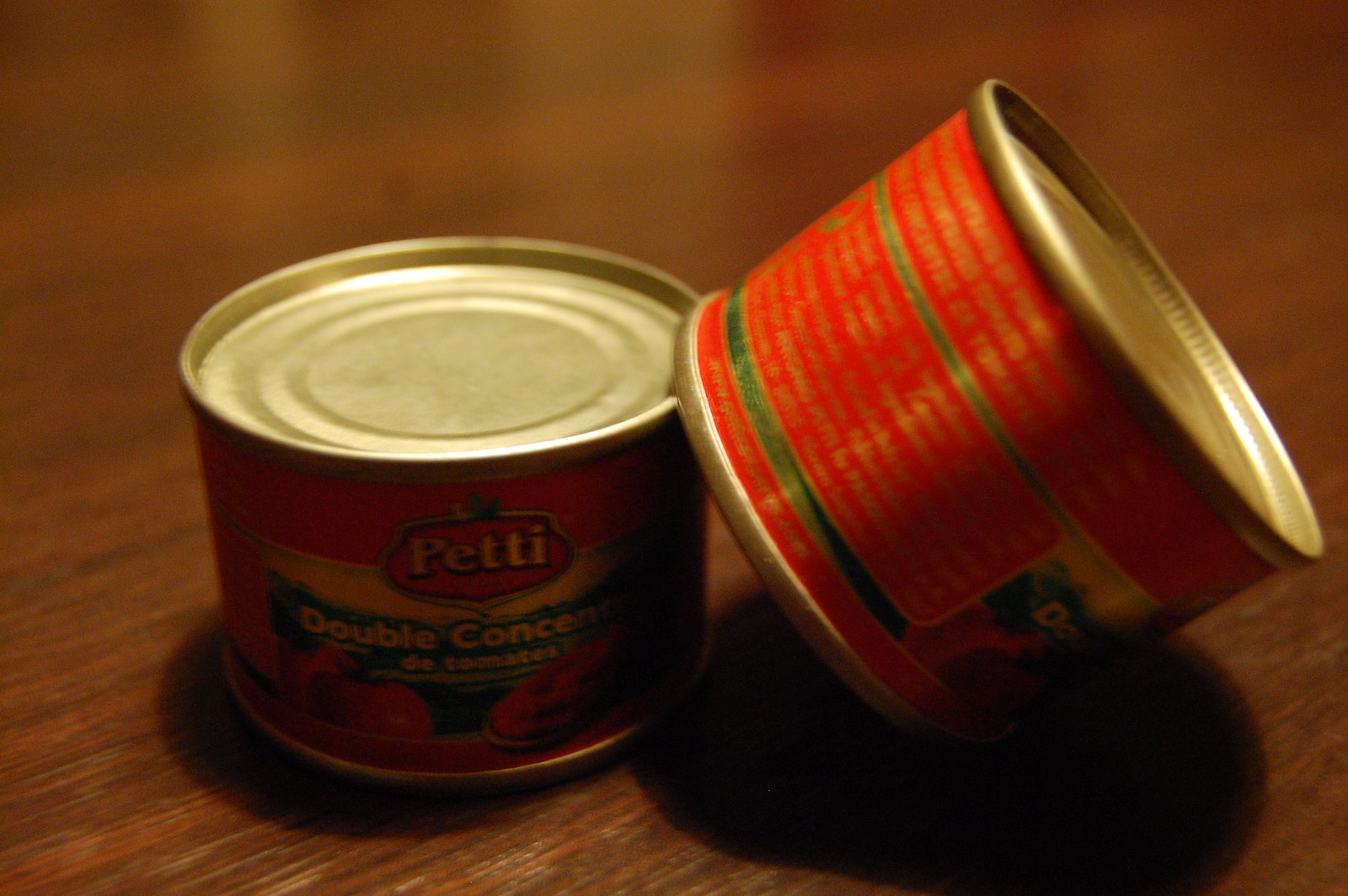The image features two small cans of tomatoes, both positioned on a shiny wooden surface, likely a table. The cans, similar in size, appear to be about four ounces each. One can is standing upright on the table, while the other is tilted to the right, with its base partially resting on the upright can and the table. The label on the upright can is fully visible, highlighting a red emblem or shield that reads "Petti" in white letters. Beneath this, the label indicates "double concentrate of tomatoes" along with images of tomatoes, suggesting tomato paste or sauce. The second can, though slightly blurred and difficult to read, appears to have a red label with some gold text. The tilted can has a gold lid, adding a touch of contrast to the scene.